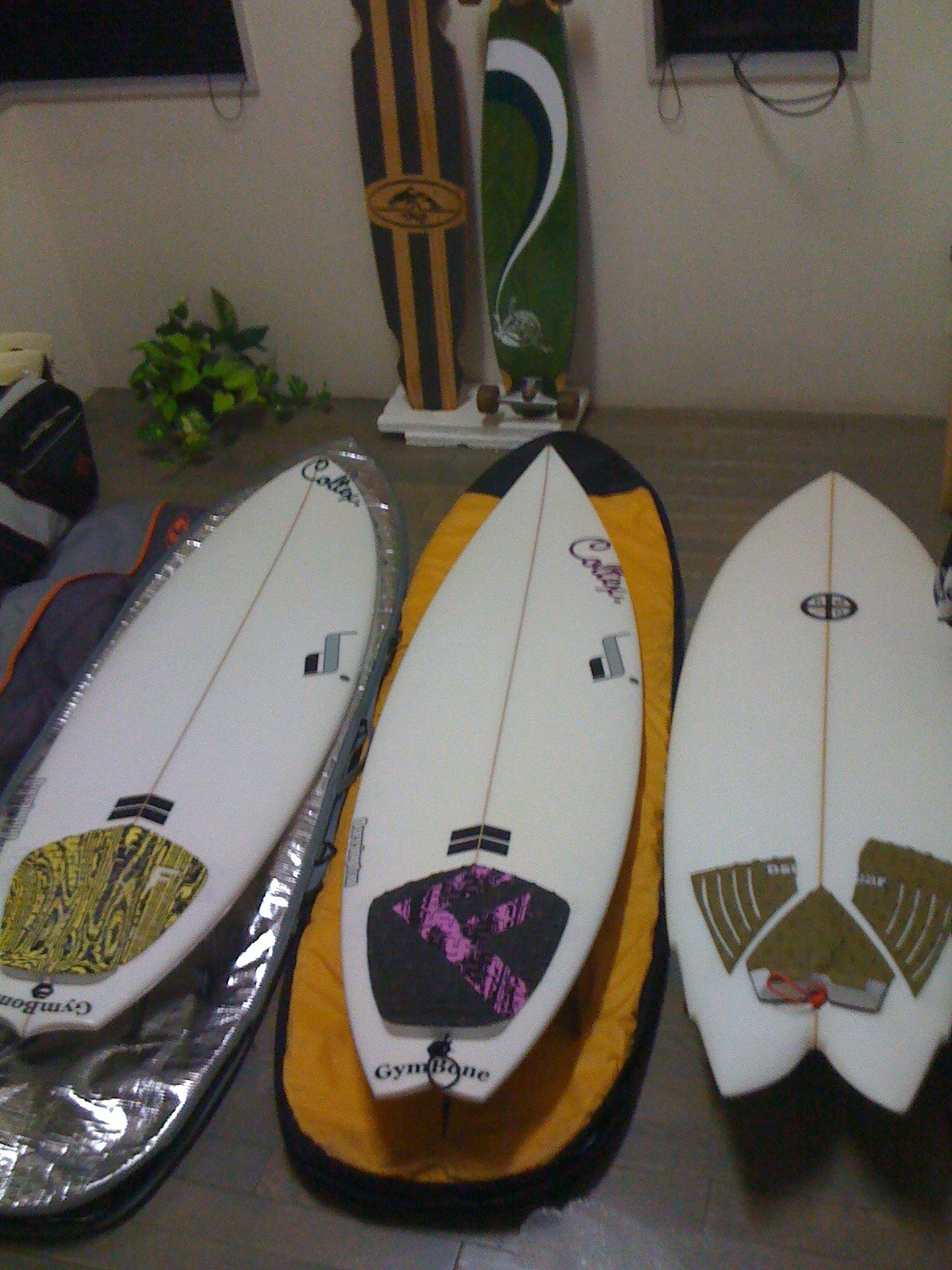This photograph features an array of surfboards and boogie boards meticulously arranged on a dark gray concrete-like surface. In the foreground, three white surfboards are stacked horizontally, each displaying unique patterns at their ends: a yellow and black design on the leftmost board, a purple and black motif on the center board, and a brown and white pattern on the rightmost board. The surfboards rest on protective sleeves, with the leftmost one on a silver foil-like cover and the center one on an orange cover. 

To the back left, a green potted plant adds a touch of nature to the scene. Leaning against the wall in the background are two more upright boards: one features black and white stripes while the other is green with a wavy white stripe and appears to have wheels—implying it could be a skateboard. The setting includes visible elements such as two windows with wires extending out and a wooden structure, possibly a storage area, enhancing the overall sense of an organized, yet lived-in space.